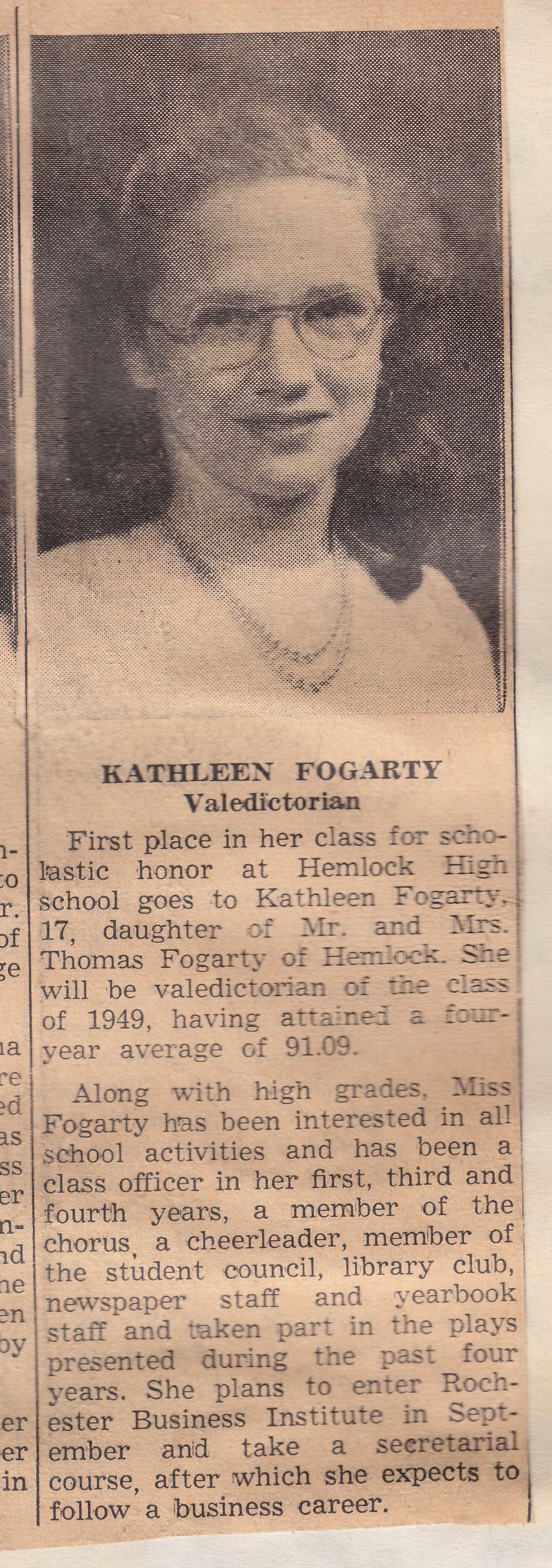This vintage black-and-white newspaper clipping presents a portrait of Kathleen Fogarty, valedictorian of the Hemlock High School class of 1949. The image, which appears at the top of the one-column article, shows Kathleen smiling and looking upward. She wears wire-rimmed glasses, a white top, and a two-strand pearl necklace, with her long, curly hair pulled back. The text beneath the portrait reads, "Kathleen Fogarty, valedictorian."

The article highlights that Kathleen, age 17, is the daughter of Mr. and Mrs. Thomas Fogarty of Hemlock. She achieved the highest scholastic honor in her class with a four-year average of 91.09. In addition to her outstanding academic record, Kathleen has been actively involved in various school activities. She served as a class officer during her first, third, and fourth years and participated in the CHORUS, Student Council, Library Club, newspaper staff, yearbook staff, and as a cheerleader. She also took part in school plays throughout her high school years. Kathleen plans to attend Rochester Business Institute in September to take a secretarial course, aspiring to pursue a career in business.